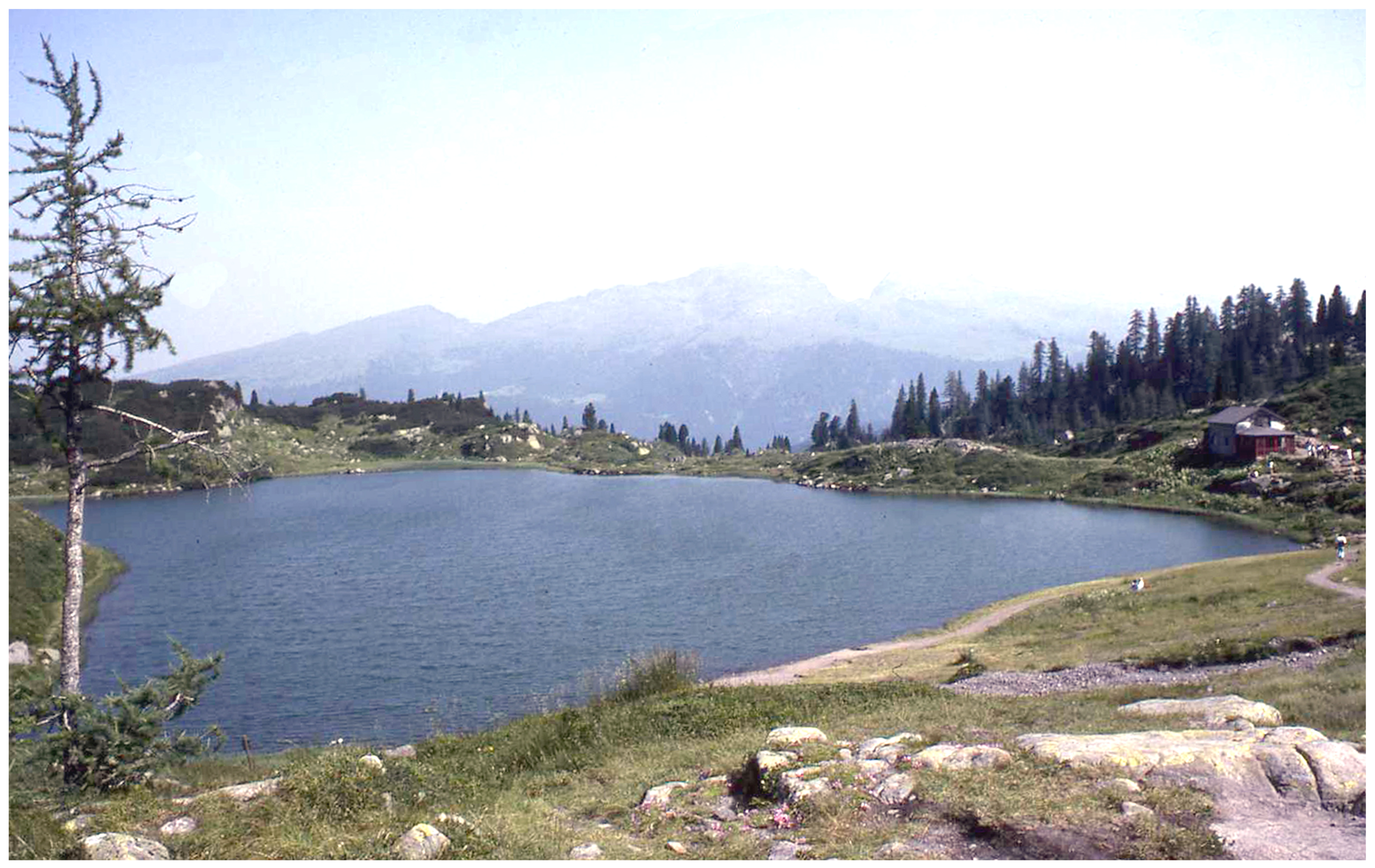This picturesque outdoor image captures a serene landscape dominated by a large, tranquil lake bordered by vibrant green grass. A charming cabin with a gray roof sits quietly on the right side of the lake, nestled in front of a dense forest of trees. To the left, a lone tree with sparse branches stretches upwards, almost reaching the top of the image. Scattered rocks and a dirt path add texture to the lush greenery surrounding the lake. The background features majestic mountains, slightly obscured and washed out by the bright, nearly cloudless sky, which fades from a striking blue to almost white at the top due to the intense sunlight. The entire scene exudes a peaceful, almost village-like atmosphere that evokes the idyllic settings of Eastern Europe, likely captured during the spring or summer months.